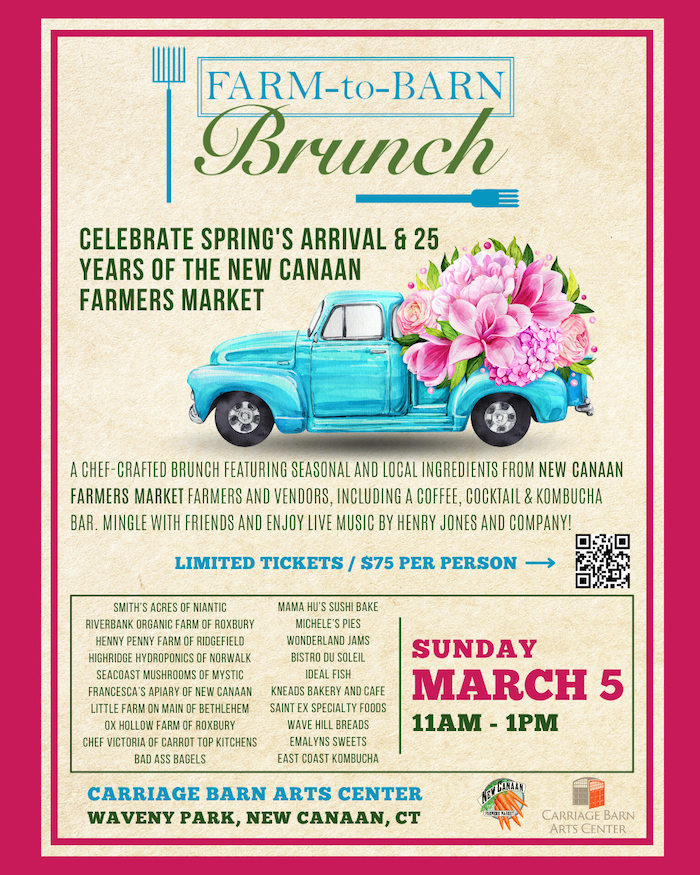The flyer for the Farm to Barn Brunch event is a rectangular poster with the left and right sides twice as long as the top and bottom sides. The poster features a thick purple border on all four sides followed by an inner, thinner purple border against a tan-colored background.

At the top of the poster, in blue text, it reads "Farm to Farm Brunch," with "Brunch" highlighted in green text. An illustration of a rake is positioned to the left of the title. Below this, in green text, it states "Celebrate Spring's Arrival and 25 Years of the New Canaan Farmers Market."

A central illustration showcases a classic 1940s blue pickup truck carrying large pink flowers in its bed. Below the truck, text describes the event as a chef-crafted brunch featuring seasonal and local ingredients from the New Canaan Farmers Market. Attendees can enjoy offerings from farmers and vendors, including a coffee, cocktail, and kombucha bar. The event encourages mingling with friends and enjoying live music by Henry Jones and Company.

Details include limited tickets priced at $75 per person, with mention of various vendors such as Smith's Acres of Niantic, Riverbank Organic Farm of Roxbury, Henny Penny Farm of Richfield, and High Ridge Hydroponics of Norfolk. Additionally, the Carriage Barn Art Center is listed as the event location, which is scheduled for a Sunday in March from 11 a.m. to 1 p.m. The flyer also features a QR code for purchasing tickets.